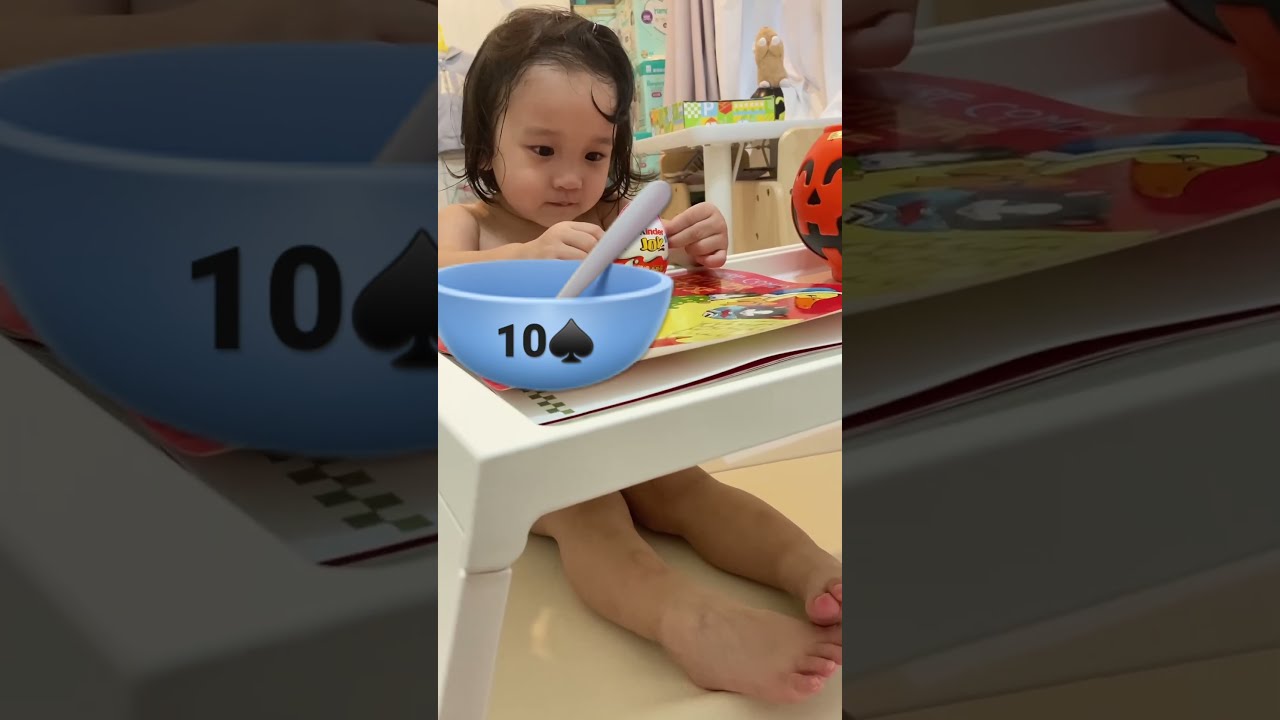In this image, a young child, possibly a toddler, is seated at a white plastic tray table which reaches just under their neck. The child has longish brown hair with a slight curl on the right side of their forehead. In front of the child is a large, powder blue bowl featuring a black spade and the number 10. A silver spoon is placed inside the bowl. The child appears to be intently focused on an activity paper or toy game also on the table. To the right of the child, there is a plastic jack-o'-lantern pumpkin, reminiscent of those used during trick-or-treating.

The background includes shelving with indistinguishable items and possibly another white table. There are pink drapes that suggest the setting might be a nursery or daycare. The image appears to be captured in the aspect ratio of a smartphone, indicating it might be a screenshot from a video. Overall, the scene depicts a young child engaged in play or an activity, surrounded by objects that add a touch of seasonal decor.